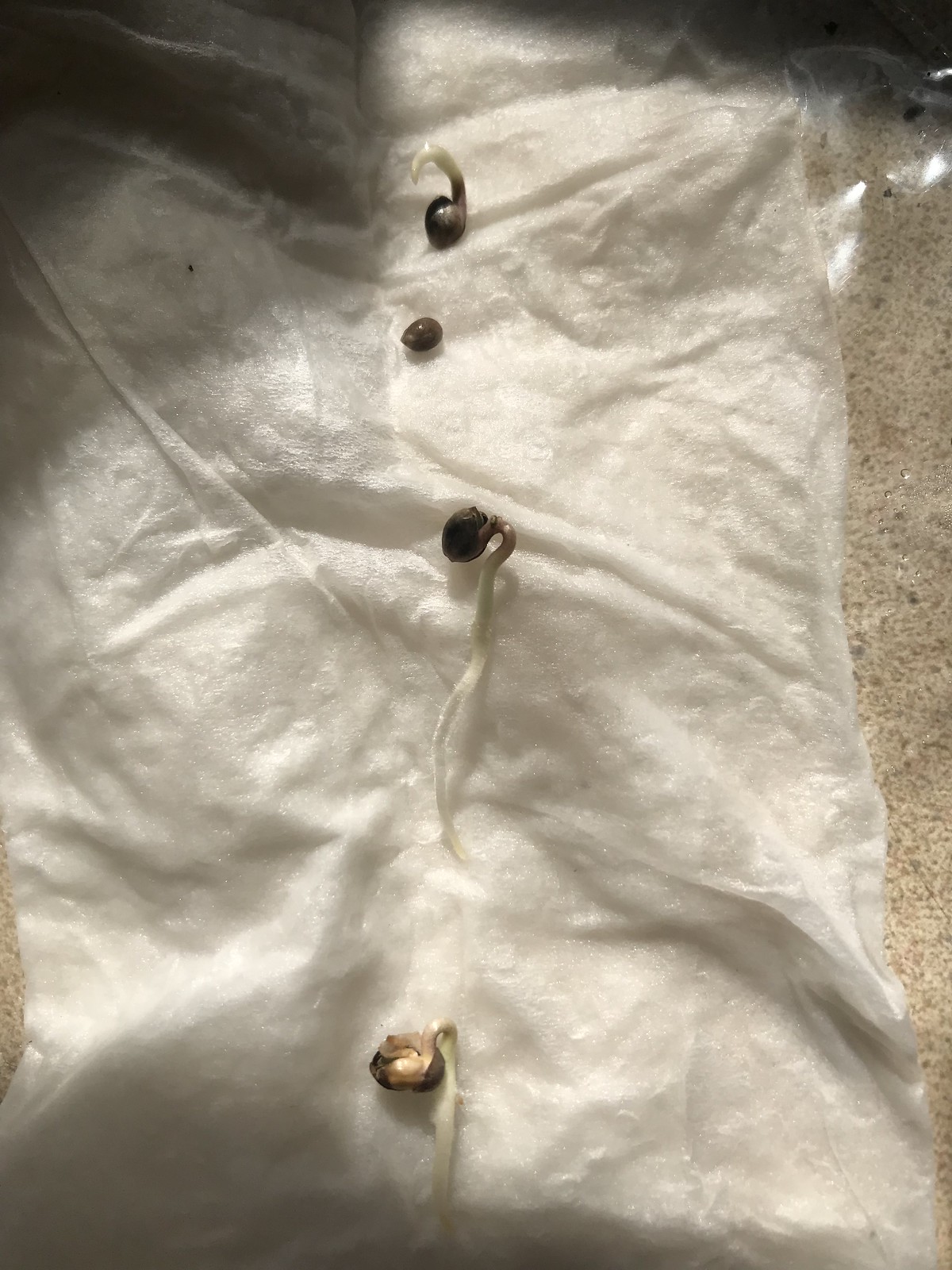The image depicts a white, shiny, crinkled material, resembling a piece of tissue paper or a wet paper towel, laid out on a white countertop or base tile to the right. On the material, several small brown elements are present, each with white root-like structures emerging from them. These elements resemble budding seeds at various stages of sprouting. The central seed has a relatively long white root, while another one nearby has a shorter root, still in the initial growth phase. Additional seeds can be seen, where the top one shows early signs of a budding root, whereas the bottom seed is less developed. Overall, the scene seems to capture sprouting seeds collected on the tissue paper.